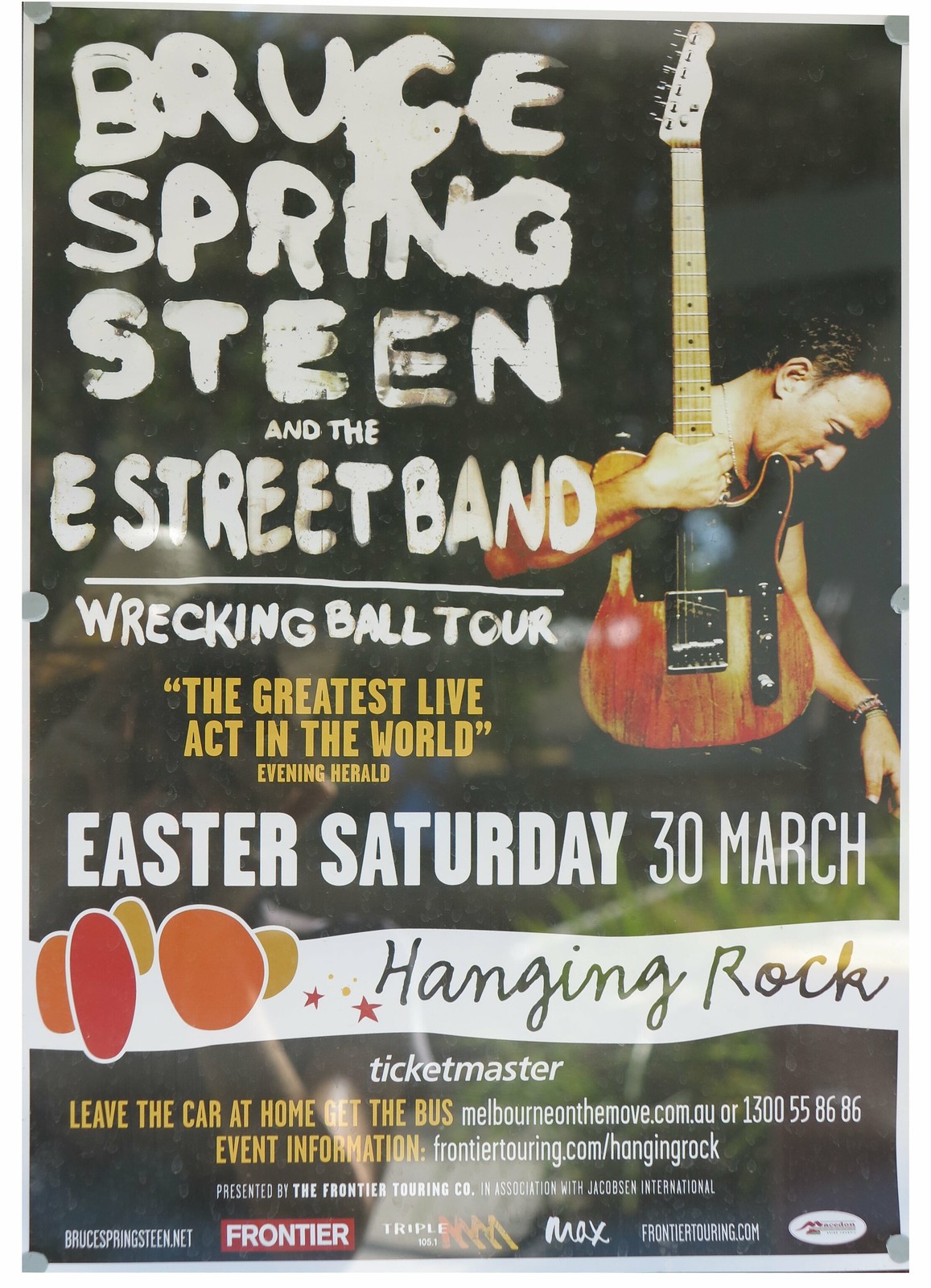This vibrant, portrait-oriented poster advertises the Bruce Springsteen and the E Street Band's Wrecking Ball Tour. The design, a blend of color photograph and graphic typography, prominently features a photograph of Bruce Springsteen on the top right. With light skin and dark short hair, he is depicted in profile, looking down, and holding a classical guitar in his left hand while wearing a black shirt and a bracelet. The top left of the poster, adorned in handwritten lettering, reads "Bruce Springsteen and the E Street Band," followed by the tour title "Wrecking Ball Tour." A striking yellow quote below heralds them as "The Greatest Live Act in the World." Event details highlight "Easter Sunday, 30 March" in bold white, with a curvy white banner underneath intricately marked "Hanging Rock" in black script, flanked by yellow, red, and gold ellipses. At the bottom, the Ticketmaster icon provides ticket information alongside additional event details and sponsor logos, urging attendees to "Leave the car at home, get the bus." This captivating poster, presented by the Frontier Touring Company, embodies the energy and excitement of the highly anticipated concert.